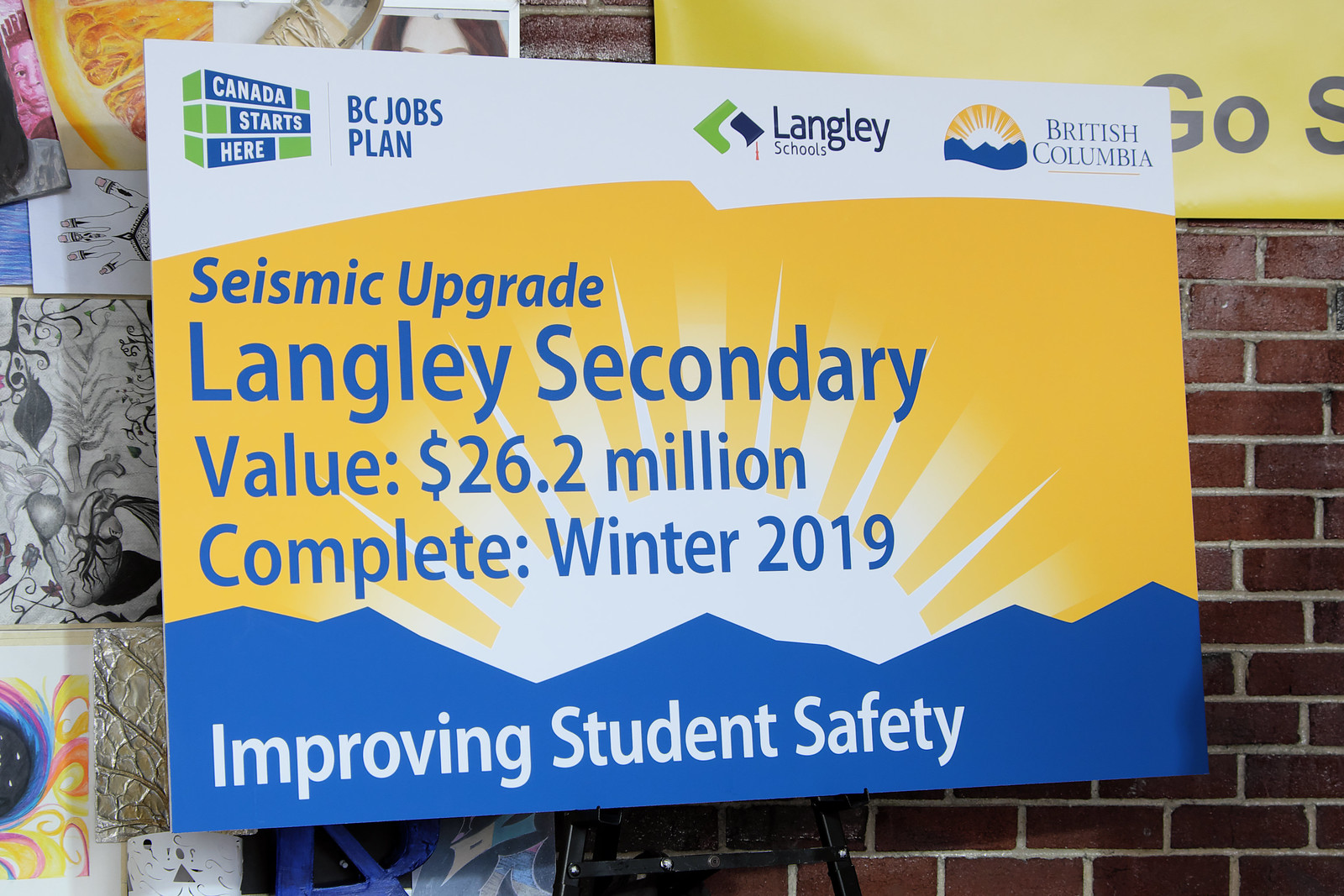The image showcases a rectangular sign mounted on a sign holder in what appears to be a school or office setting, positioned against a red brick wall with white mortar. Behind the main sign, there is another yellow sign affixed to the wall and several student-made drawings. The central poster is predominantly yellow and blue, featuring a design with a sun and blue mountains against a white sky border. The sign prominently reads "Canada Starts Here, BC Jobs Plan, Langley Schools, British Columbia." It announces a "$26.2 Million Systematic Upgrade to Langley Secondary" and notes its completion date as "Winter 2019," additionally highlighting its achievement as the "Winner of 2019 Improving Student Safety."